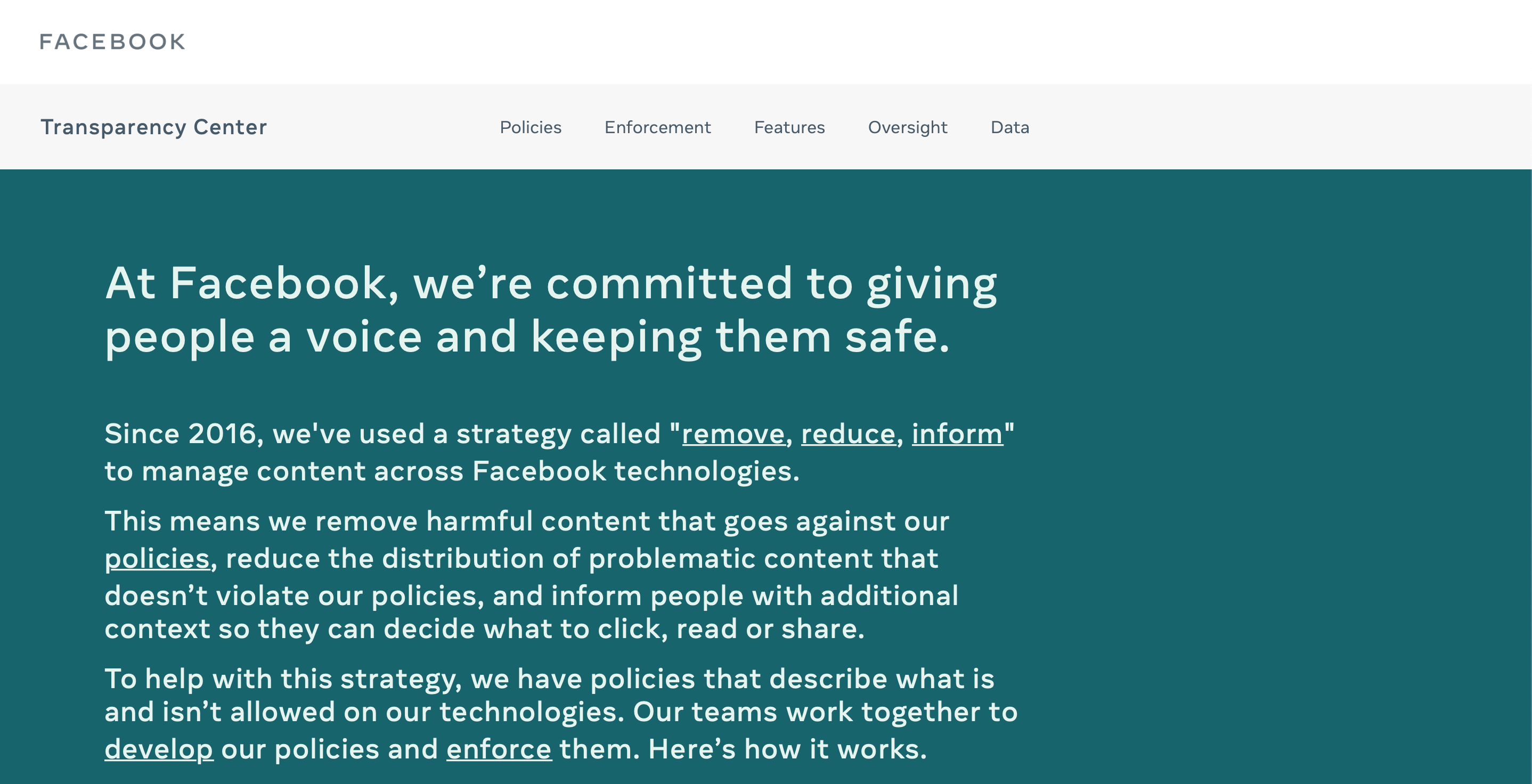This image is a detailed infographic from Facebook, focusing on their Transparency Center. The main section presents Facebook's commitment to balancing the provision of a voice for users with ensuring their safety. Key text on a dark green background with white lettering states, "At Facebook, we're committed to giving people a voice and keeping them safe. Since 2016, we've used a strategy called 'remove, reduce, and inform' to manage content across Facebook technologies."

The text further explains the strategy:
- **Remove** harmful content that violates policies.
- **Reduce** the distribution of problematic content that doesn't necessarily violate policies.
- **Inform** users with additional context so they can make informed decisions about what to click, read, or share.

Supporting this strategy are policies detailing allowable and prohibited actions on Facebook's services. Their teams collaboratively develop and enforce these policies.

The image design includes a white header with the Facebook logo, followed by a gray strip featuring the Transparency Center and navigation links. The main content area is highlighted against a dark green background with all text left-justified, leaving significant negative space on the right side, maintaining a balanced visual aesthetic.